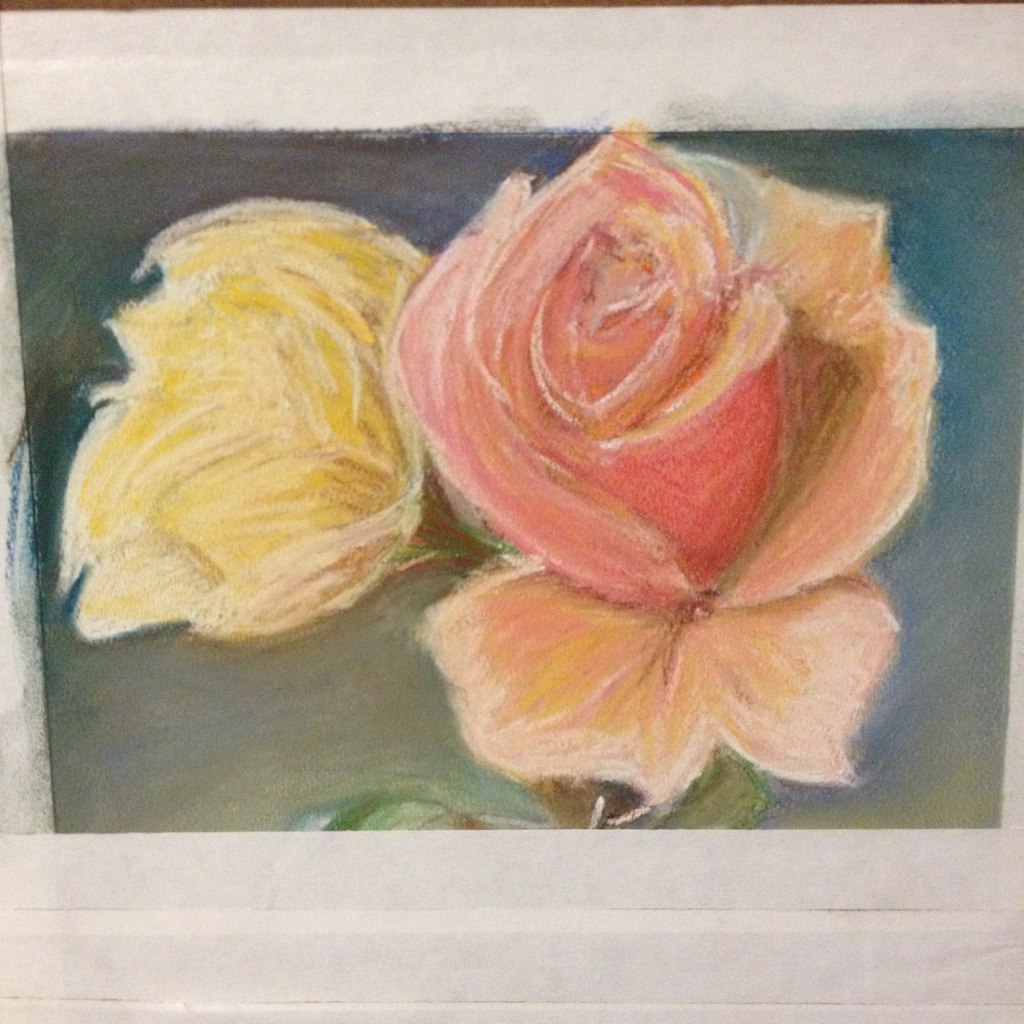The artwork showcases a vividly detailed, colored pencil and pastel drawing of two flowers on a white canvas. Dominating the right side of the composition is a large, partially closed rose, with petals shifting from a rich, reddish core to orangish and pinkish hues towards the edges. Adjacent to it on the left is a smaller, predominantly yellow flower, resembling a carnation. Both flowers are anchored by a stem adorned with green leaves. The backdrop of the image transitions from a dark, muted blue and green at the top to a lighter, more grayish tone at the bottom, imparting a textured, almost fluid quality to the entire piece. Notably, the coloring of the background and the flowers is somewhat faded and loosely rendered, giving an impressionistic feel with visible lines and powdery shading. The borders of the drawing are also irregular, reflecting a spontaneous and expressive artistic technique. Overall, the piece exudes a sense of connectedness to the artist’s emotional expression, with highlighted spots of white and dark brown adding depth and contrast.